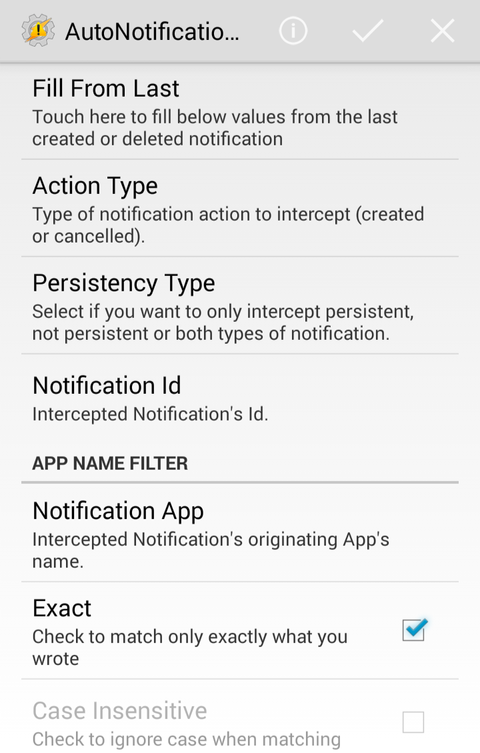The image appears to be a screenshot from a mobile phone, featuring a user interface for managing notifications. At the very top, a gray border spans the width of the image, with a gray gear icon containing a black exclamation mark to the left side, accompanied by the text "Auto Notification...". To the right of this icon, there are three symbols: a white circle with an "i" inside, a checkmark, and an "X."

Below the top section, the background transitions to gray, displaying four sequential options:

1. **Fill from Last**: A prompt that reads, "Touch here to fill below values from the last created or deleted notification."
2. **Action Type**: A section explaining, "Type of notification action to intercept: created or canceled."
3. **Persistency Type**: Instructions to "Select if you want to only intercept persistent, non-persistent, or both types of notifications."
4. **Notification ID**: Simple text stating "Intercepted notification's ID."

Further down, there is a heading titled **App Name Filter**. Below this heading are two options:

1. **Notification App**: Describes "Intercepted notification's originating app's name."
2. **Exact**: Indicates "Check to match only exactly what you wrote," with a blue checkmark in a box to the right of the text.

At the bottom of this section is an additional option labeled **Case Insensitive**, accompanied by a description urging users to "Check to ignore case when matching."